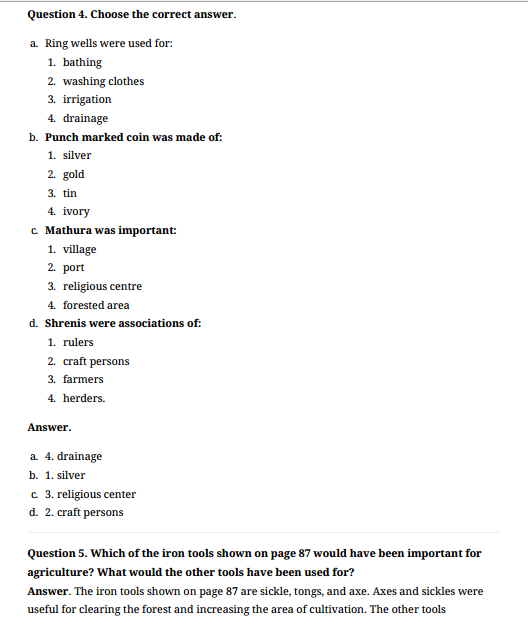The image is a screenshot featuring a white background with predominantly black text, set up in a format reminiscent of a school textbook. At the top, a thin black border frames the title which reads, "Question 4. Choose the correct answer." Below the title, a series of multiple-choice questions and their corresponding answers are presented, formatted with alphabetical labels and numerical options:

- Question A: "Ring wells were used for"
  1. Bathing
  2. Washing clothes
  3. Irrigation
  4. Drainage
  - Answer: 4. Drainage

- Question B: "Punch marked coin was made of"
  1. Silver
  2. Gold
  3. Tin
  4. Ivory
  - Answer: 1. Silver

- Question C: "Mathura was important"
  1. Village
  2. Port
  3. Religious center
  4. Forested area
  - Answer: 3. Religious center

- Question D: "Centers were associations of"
  1. Rulers
  2. Craft persons
  3. Farmers
  4. Herders
  - Answer: 2. Craft persons

Additionally, there is a "Question 5," stated in sentence form, followed by an answer directly beneath it. The clean and straightforward layout of the text resembles typical educational material.